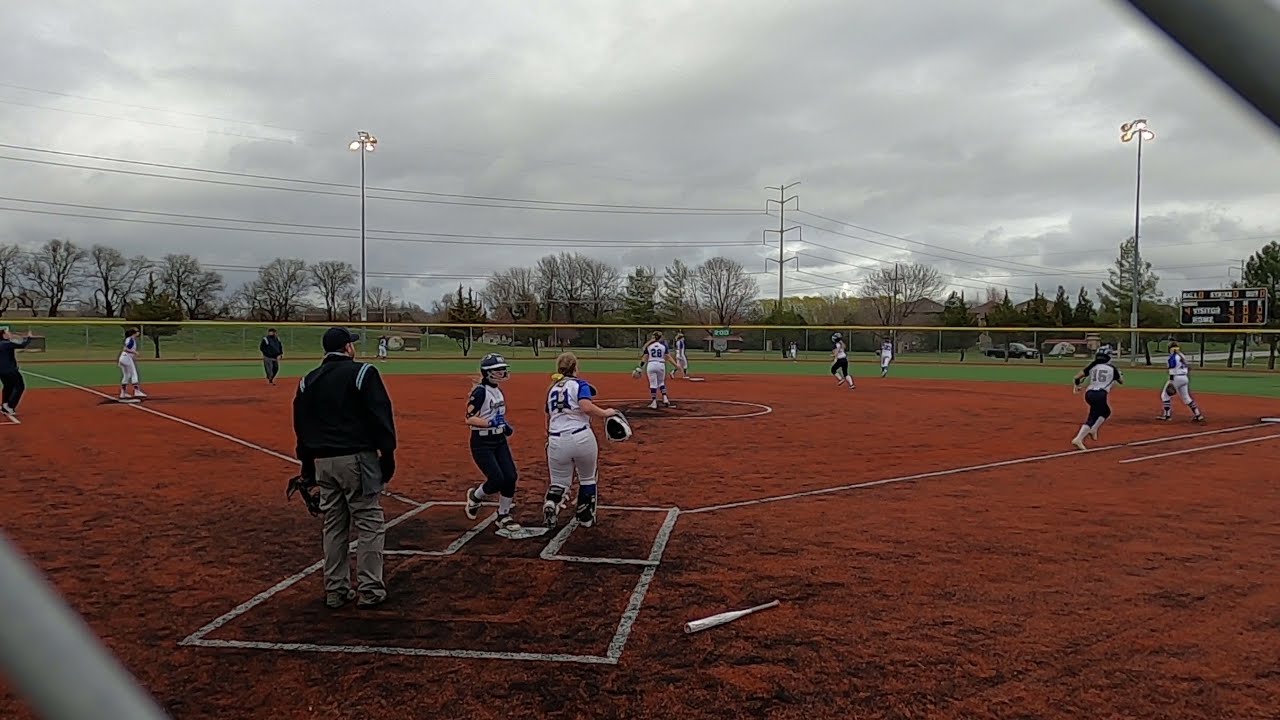The image captures a lively scene of a women's softball game in action. The softball field, outlined with white lines on a reddish-brown soil infield, extends into a lush green grass outfield. The sky is heavily overcast, casting a dim light on the field necessitating the use of tall floodlights. The presence of barren trees suggests it could be fall or winter. In the foreground, a catcher with her helmet off is seen running hurriedly towards the field, implying an ongoing play. A batter is sprinting towards first base while another player appears to have just scored a run. The rest of the players are in their usual positions, with some facing away from the camera, focused on the ball's trajectory. On the periphery, men in grayish-brown pants and black long-sleeved jackets, likely officials or coaches, are stationed. An umpire stands vigilant behind home plate, and a bat lies abandoned to the right. The backdrop shows electrical posts and distant trees, complementing the dynamic energy of the game despite the somber, cloudy sky.